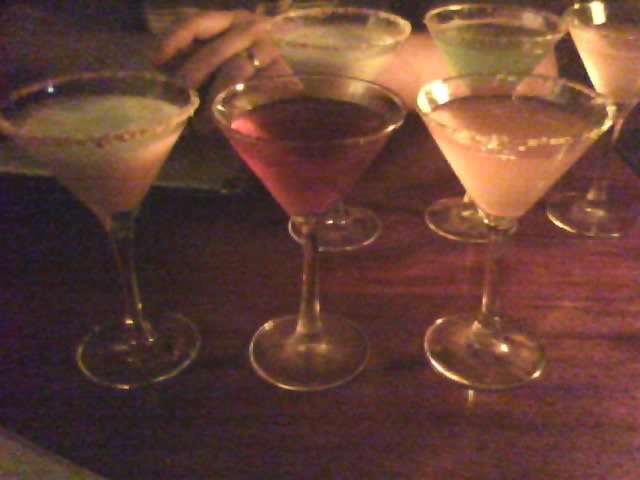In this low-light, close-up image, we see six martini glasses arranged on a smooth, glossy medium-brown wooden tabletop. Each glass holds a different colored liquid, adding a vibrant contrast to the subdued background. The drinks, featuring a variety of hues—white, deep red, pink, light green, dark green, and purple—suggest multiple flavors, each with rims adorned in salt or sugar. The martini glasses, with their characteristic upside-down bell shape, long stems, and round bases, display a hint of peach salt around one rim, heightening the sensory detail. In the background, partially in the frame, is a man's folded arm resting on the table, his gold wedding band clearly visible, hinting at a social gathering, possibly in a restaurant setting. The photo’s slight fuzziness and dim lighting evoke a casual, intimate ambiance.